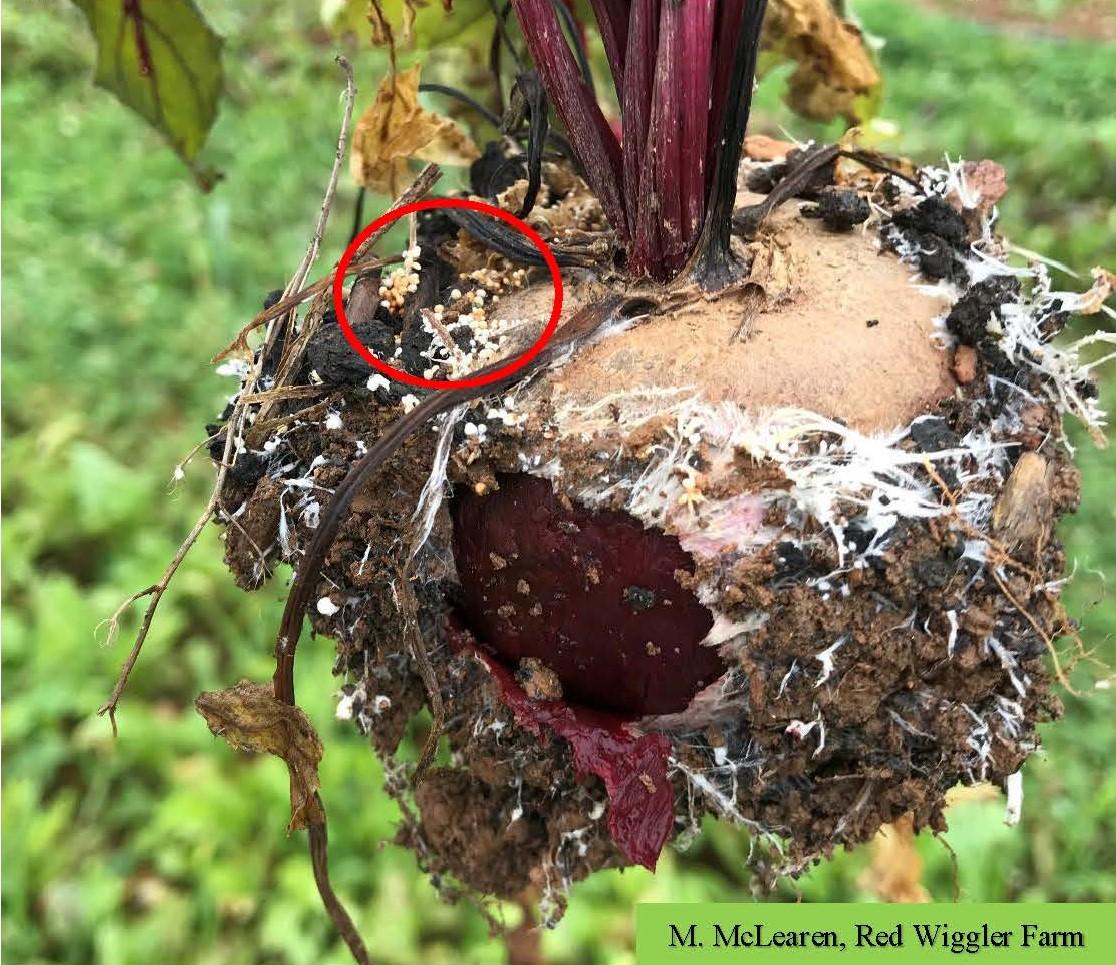This detailed photograph from "M. McLaren Red Wiggler Farm" primarily features a pulled-up plant root, zoomed in to show extensive detail. The root, quite large and round, is held up by a person and appears very dirty, with an exterior covered in white patches while the interior reveals a reddish color. The image is bordered with a green box featuring black text identifying the source. A red circle is drawn on the top left portion of the root, highlighting small, white, round balls that may be Wiggler eggs or some type of fungal growth. Pinkish-red roots extend from the object, which is surrounded by blurred foliage and grass in the background. The entire scene suggests a farm dedicated to cultivating or researching these Wigglers.